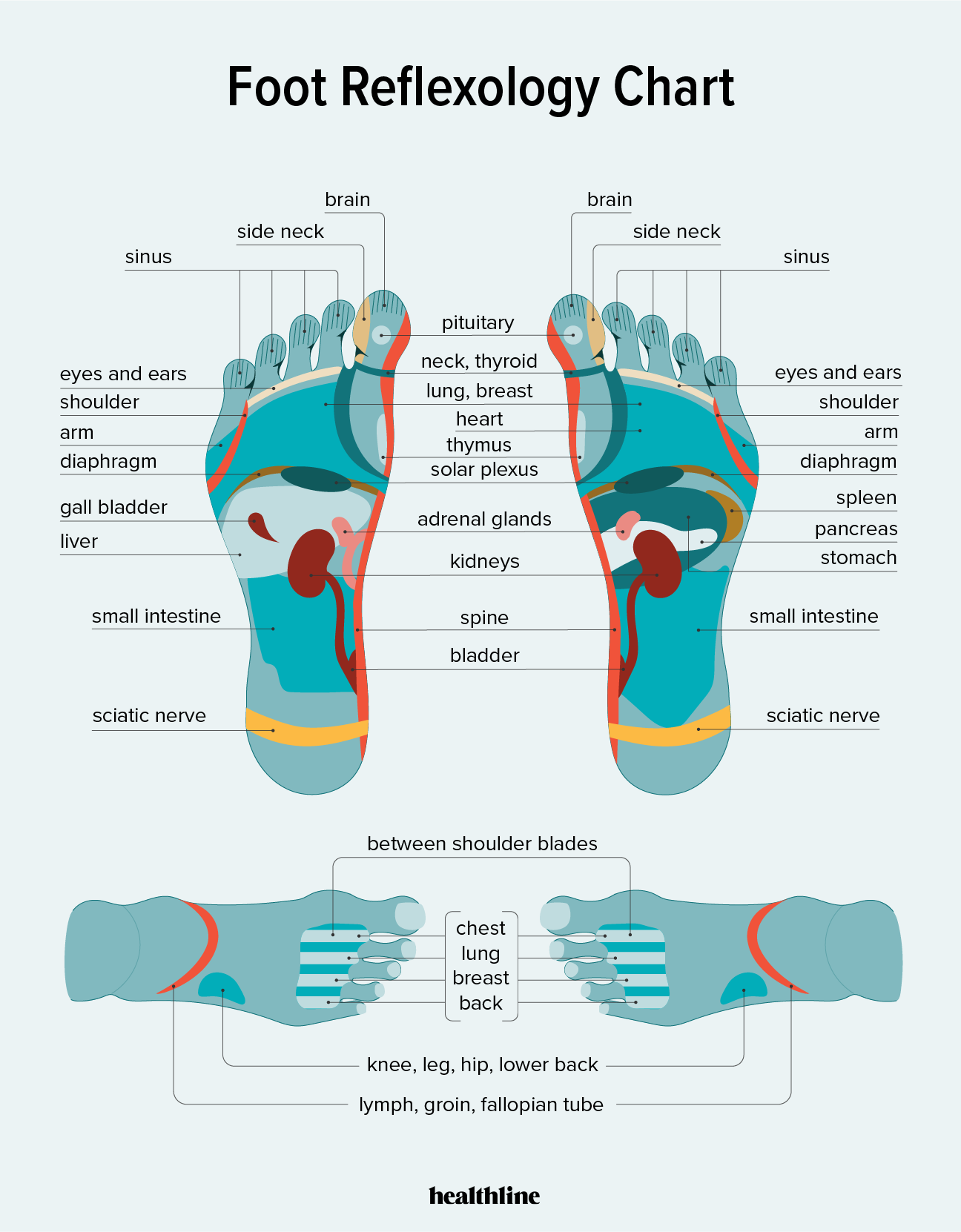The "Foot Reflexology Chart" is a detailed Healthline illustration designed to map out various parts of the body as they correspond to specific areas of the feet. At the top of the chart, the title is prominently displayed in black text. Directly underneath, the chart features hand-drawn illustrations of a left and right foot, showcasing their soles with various body parts labeled and color-coded. These labels include the brain, side neck, sinus, eyes and ears, shoulder, arm, diaphragm, gallbladder, liver, small intestine, sciatic nerve, pituitary, neck, thyroid, lung, breast, heart, thymus, solar plexus, adrenal glands, kidney, spine, bladder, and more. Towards the bottom of the chart, there are additional illustrations of the feet facing each other, highlighting areas associated with the chest, lung, breast, and back. The feet illustrations are colored in shades of light blue, teal, orange, yellow, pink, and red to differentiate the various areas, making the chart visually engaging and easy to interpret. At the very bottom, "Healthline" is printed in bold black text, signifying the source of the illustration.